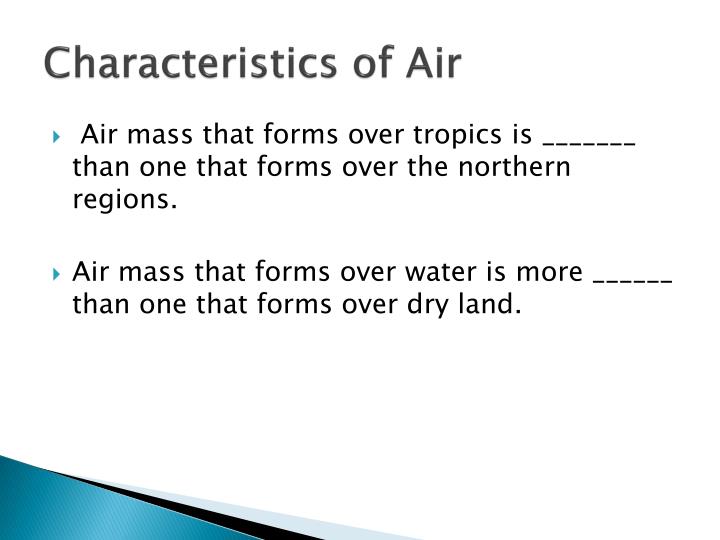This image depicts a PowerPoint slide titled "Characteristics of Air." Under this heading, there are two bullet points marked by small blue triangles. The first bullet point states, "Air mass that forms over tropics is ______, then one that forms over the northern regions," highlighting a need to fill in the blank during the presentation. The second bullet point reads, "Air mass that forms over water is more ______ than one that forms over dry land," again indicating a blank to be filled in. In the bottom left corner of the slide, there is a complex pattern consisting of three overlapping triangles: a prominent blue right-angled triangle with hints of white in its middle, a narrow black triangle extending downwards from near the top of the blue triangle, and a light blue triangle positioned above the black triangle. The base lengths of these three triangles form a horizontal alignment.